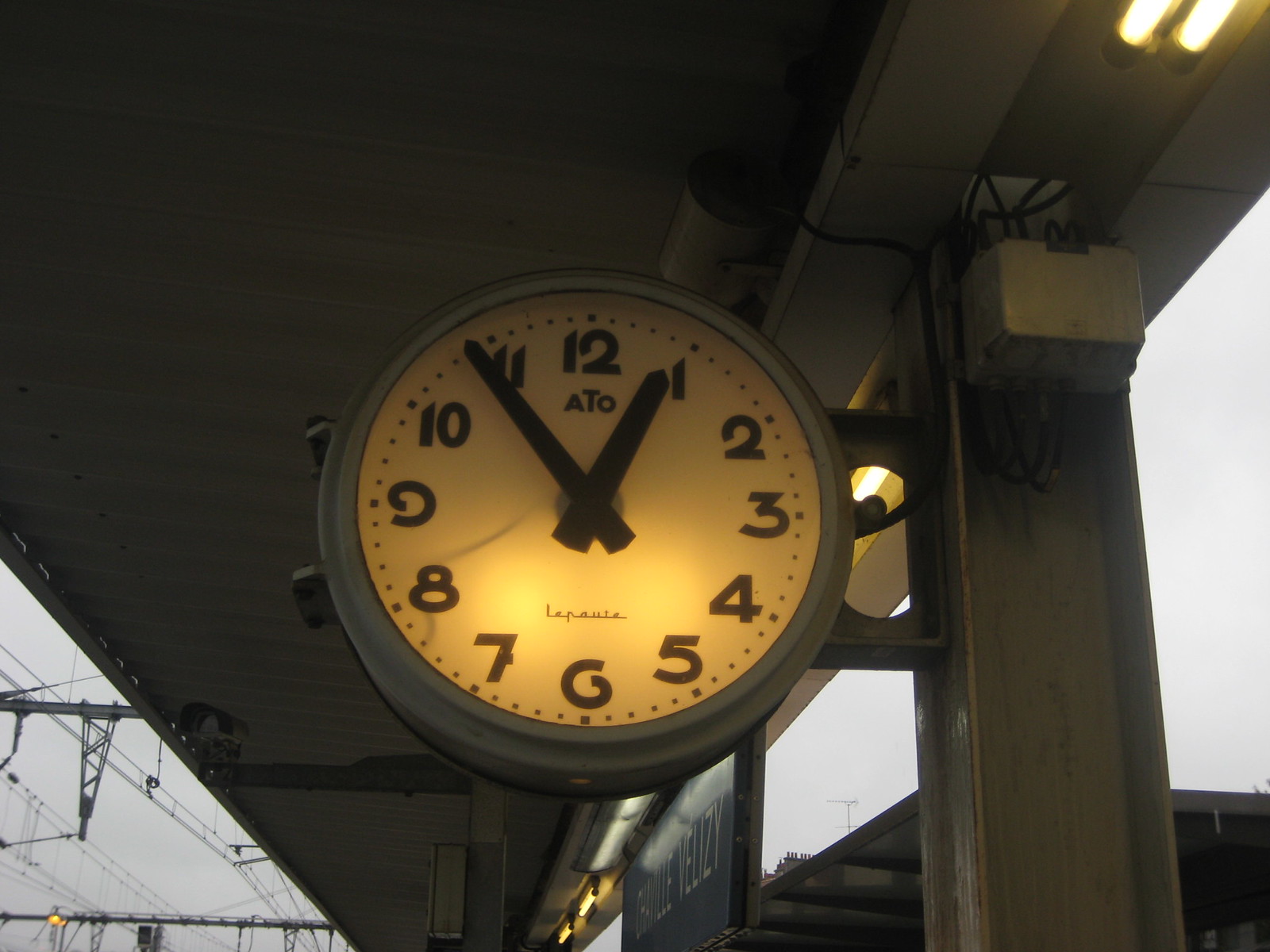The photograph features a prominently displayed silver circular clock, likely mounted outside a station. The clock, which has bold black hands and large black numerals, is illuminated by a gentle amber light that enhances its white clock face. To the left of the clock, there is a square box affixed to a pole with several black cords extending from it. The background reveals a complex metal scaffolding structure adorned with various lights and a metallic object suspended from it. Beneath the clock, there is a partially visible gunmetal-colored sign with white lettering. The scene is set against a sky blue backdrop, with the top of a distant building visible on the horizon.